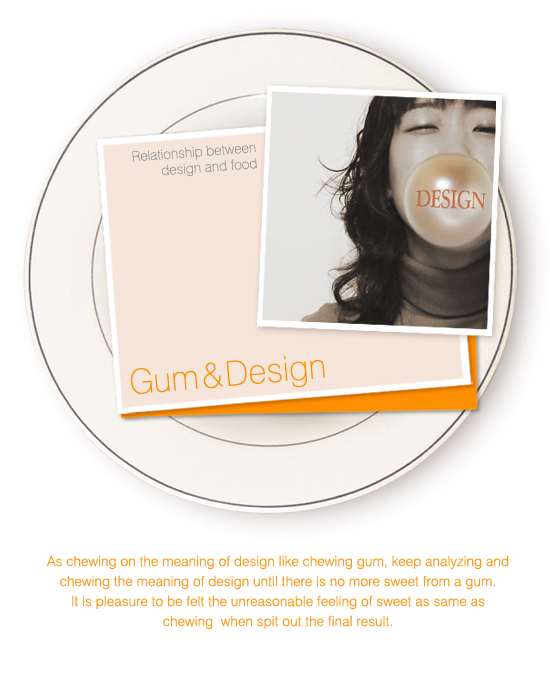The image is an advertisement for a company called "Gum and Design," focusing on the relationship between design and food. At the center of the image, there's a photograph of a woman with long, dark hair, wearing a turtleneck, and blowing a bubble made of gum. The bubble, with the word "DESIGN" written on it in orange, prominently floats in front of her closed eyes. The woman's black-and-white picture rests atop a small card that features an orange background. This card reads "RELATIONSHIP BETWEEN DESIGN AND FOOD" at the top and "GUM AND DESIGN" at the bottom in orange font. Both the photograph and the card are placed on a white, round dinner plate, viewed from above. Below the woman’s image, in orange text, the caption elaborates: "As chewing on the meaning of design like chewing gum, keep analyzing and chewing the meaning of design until there is no more sweet from a gum. It is pleasure to be felt, the unreasonable feeling of sweet as same as chewing when spitting out the final result." The entire composition symbolizes the process of savoring design much like the experience of chewing gum, blending aesthetics with a culinary metaphor.